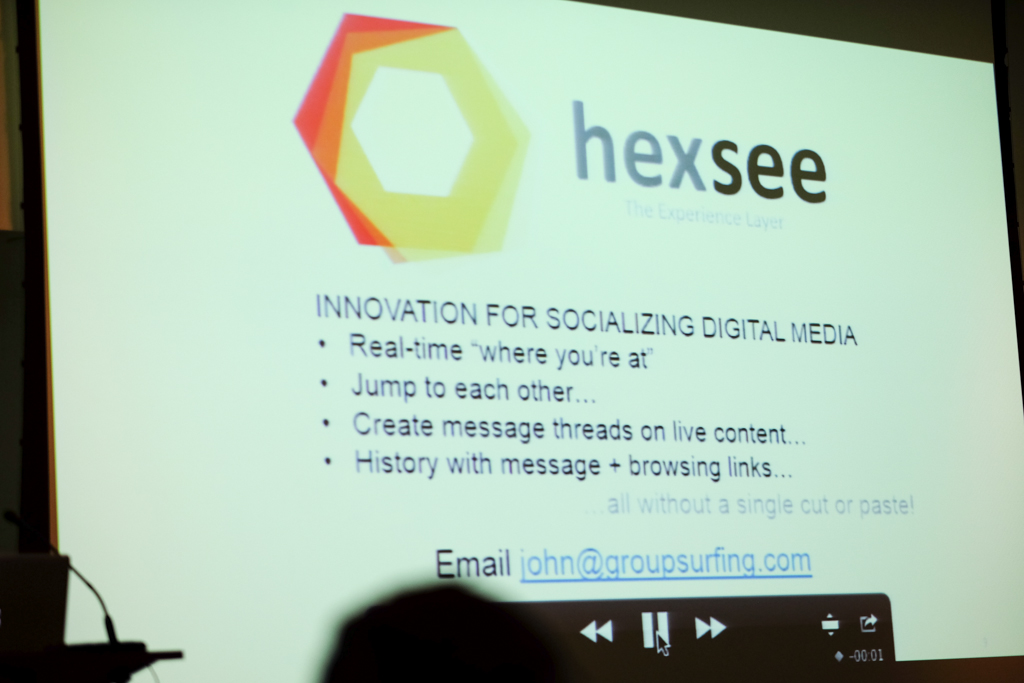The image features a close-up photograph of a large projector screen, likely taken during a lecture, conference, or class presentation. Dominating the screen is a hexagon-shaped logo that transitions in color from yellow at the center to orange and then red at the edges. To the right of this logo, the text "HEX C" is displayed, with "HEX" in blue and "C" in black. Directly below, in black text, the tagline reads "Innovation for socializing digital media." Four bullet points are listed underneath, describing: "Real-time 'where you're at'," "Jump to each other," "Create message threads on live content," and "History with message and browsing links." Additionally, an email address, "john@groupsurfing.com," is in blue text at the bottom. The screen's background is primarily white with a black bar along the top, and the shadowy outline of a podium, microphone arm, and the top of someone's head are faintly visible in the foreground, hinting at an ongoing presentation.